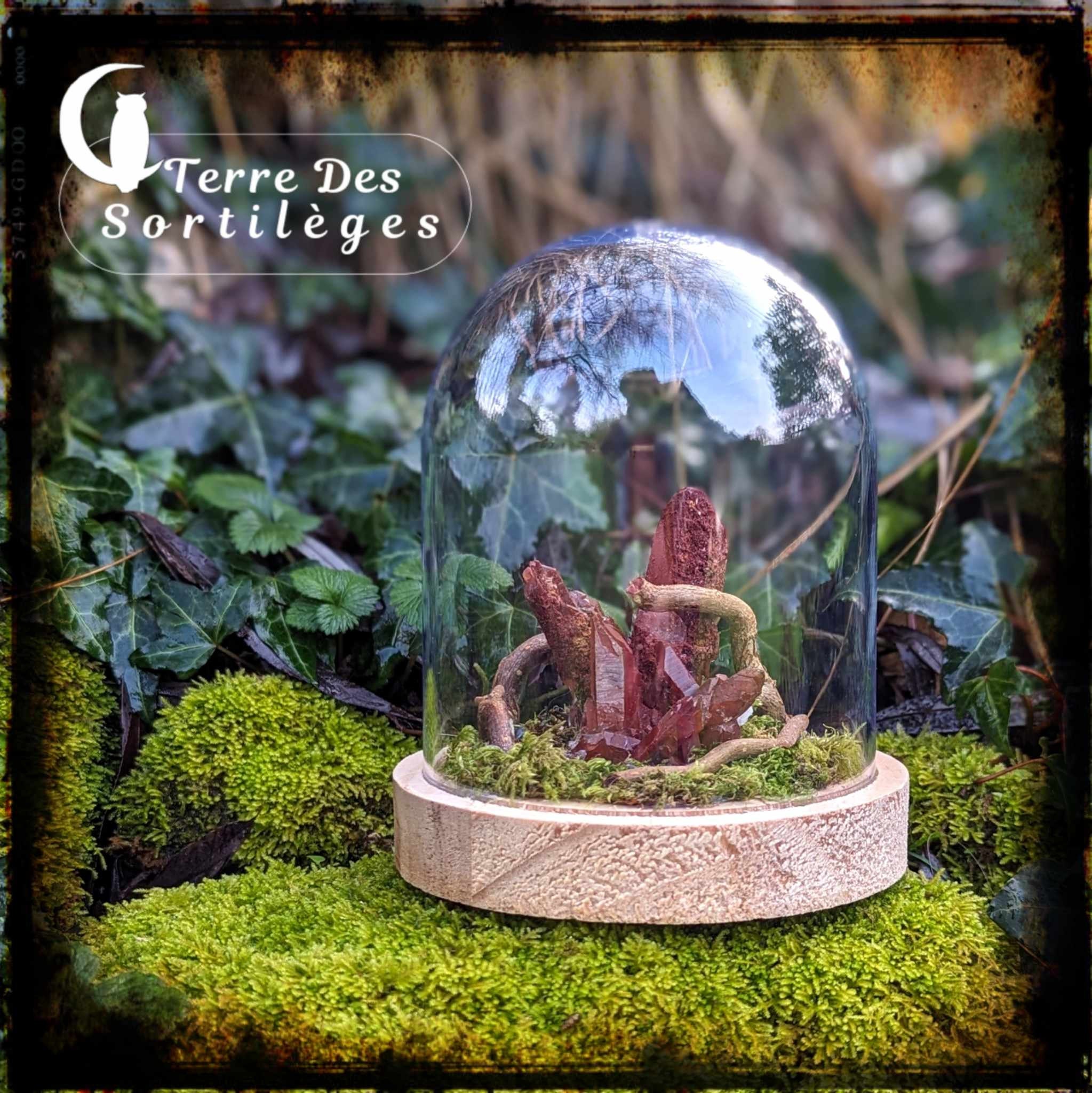The advertisement features a detailed, enchanted terrarium, resembling a snow globe. It is composed of a clear glass dome perched on a cylindrical base which appears to be made of brown cork. Inside the dome, there's a mix of intriguing elements: twisted tree trunks or brown, ruby-like crystals, and patches of green moss that add a touch of natural beauty. The centerpiece could be perceived as either a red plant or a unique crystal formation. Alongside it, slender brown branches elevate the scene, giving it an almost magical forest vibe.

The background of the image showcases a lush forest, teeming with ivy, undergrowth, and moss-covered flora. The setting is bathed in rich greenery, with the terrarium itself sitting on a vibrant patch of grass in the foreground, transitioning to more blurred, earthy tones with brown branches further back.

In the upper left corner, the logo features a crescent moon cradling an owl, above the elegant white text "Terre des Sortilèges." This French phrase enhances the mystical theme of the advertisement, harmoniously intertwining with the enchanting forest backdrop and the intricate, encapsulated world within the terrarium.